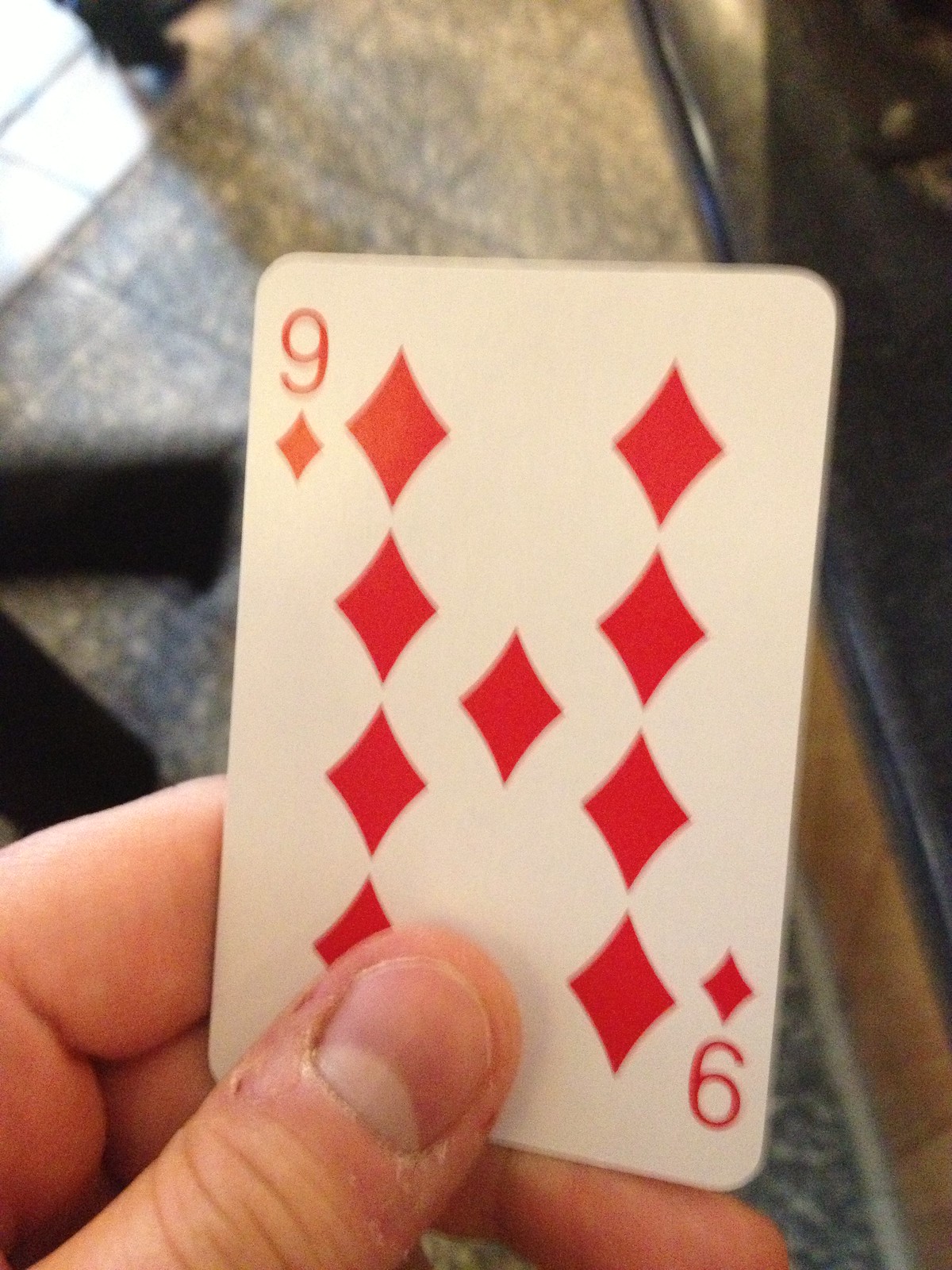A color close-up photograph features a man's left hand, showcasing his thumb, index, and middle fingers holding the Nine of Diamonds playing card. The individual has very pale skin, and the card is prominently displayed. The background reveals a floor made of beautifully variegated tiles in stone gray and golden brown hues. In the upper left corner, light streams in, likely from a nearby window, casting a natural glow on the scene. To the side, a piece of dark wooden furniture, possibly a cabinet or bookshelf, adds depth to the composition. A small sliver of hardwood flooring is visible in the bottom right corner, completing the detailed setting.